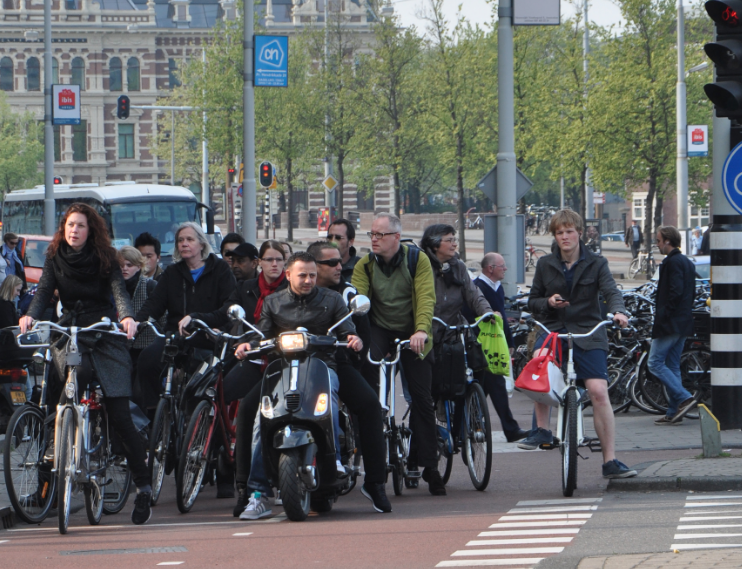The image captures a bustling city crosswalk filled with cyclists and a motorcyclist poised to cross the road. The group, viewed head-on, includes people in coats and long sweaters, some with bags hanging off their handlebars. Prominently in the foreground is a man on a motorcycle. A cyclist with a red bag on the right stands out slightly apart from the cluster. To the left, a city bus is stopped, and red stoplights signal to halt. Beyond the crosswalk, there’s a line of parked bikes and scattered pedestrians. The backdrop features a building with red and white bricks and some hanging trees. The scene is also marked by telephone poles and distinct traffic lines on the road.